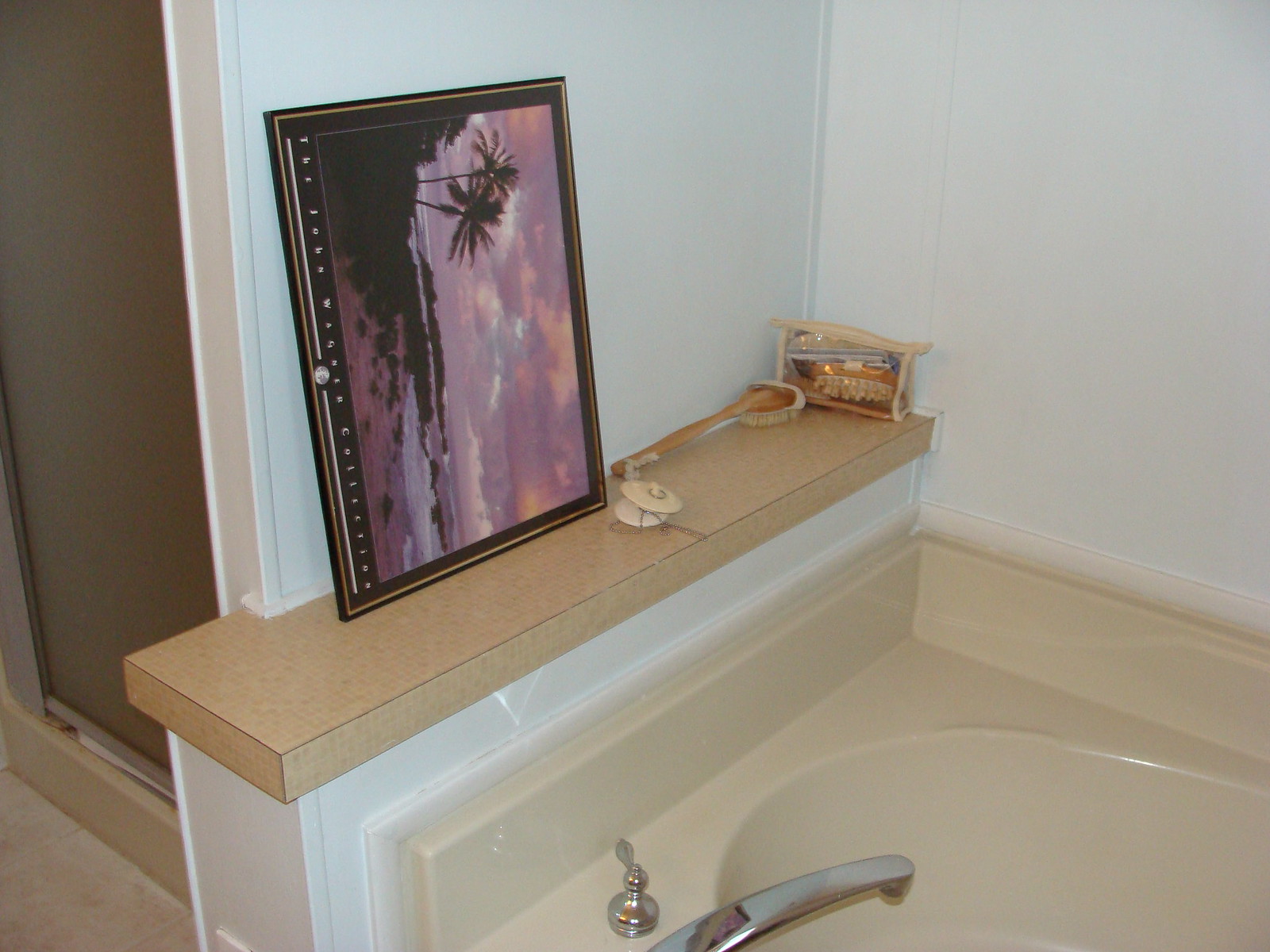The image captures a corner section of a bathroom, specifically focusing on the bathtub area. To the far left, a step-in shower is partially visible, delineated by silver metal tracking for the door. The main feature of the image is a garden tub, which appears to be from a few decades back. The tub itself is beige and not made of stone, complemented by standard silver hardware, including a spout and handle. Encircling the tub is white trim, akin to a baseboard, sealing the beige backsplash against the white bathroom walls. 

Dominating the wall to your right, facing the corner, is a slim Formica shelf in beige. Resting vertically on the shelf is a purple beach scene picture with brown palm trees, not hung as traditionally intended. The shelf also holds two tub stoppers and a bag of unspecified items. Below the shelf, an electrical outlet is noticeable. The floor is tiled in a brownish hue, adding warmth to the bathroom's color palette. The overall scene conveys a somewhat dated yet functional space.